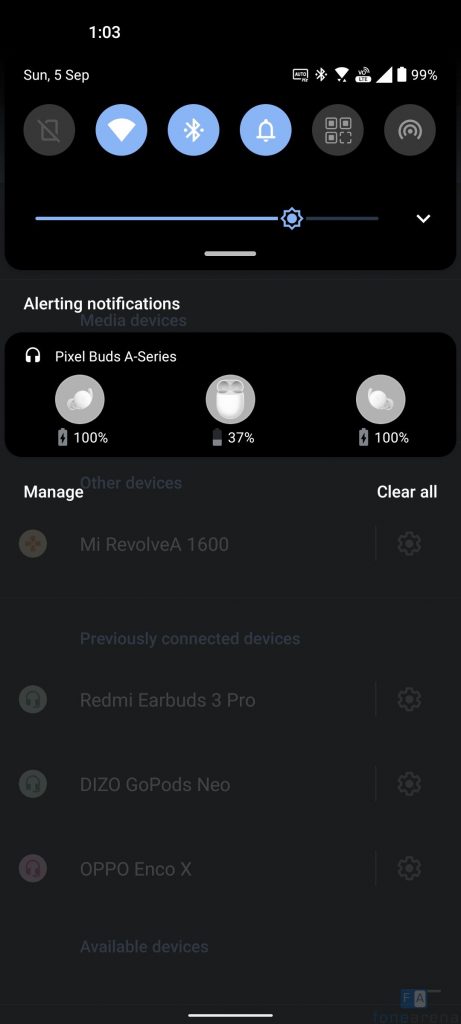A detailed screengrab of a smartphone home screen using a black theme. The top of the screen displays white text reading "10:03" on the left, with "Sunday, 5 September" directly below. On the upper-right corner are various status icons: an auto icon, Bluetooth icon, full Wi-Fi signal, LTE banner, and a battery level at 99%.

Below the time and date is a row of six circular icons. From left to right, the first icon is grayed out, followed by a blue-highlighted Wi-Fi icon, a blue-highlighted Bluetooth icon, and a blue-highlighted notification bell icon. The final two icons in the row are also grayed out. The screen brightness is set at approximately 75%.

Beneath this row, a section titled "Alerting Notifications" displays. It features the "Pixel Buds A-Series" notification with three inline icons showing battery percentages. From left to right, the icons indicate 100%, 37%, and 100%. Below this notification are options "Manage" and "Clear All."

Further down, there is a list of previously paired audio devices, shown as grayed-out settings, including various earbuds, earpods, and headphones, indicating they are no longer actively connected but still registered in the phone's settings.